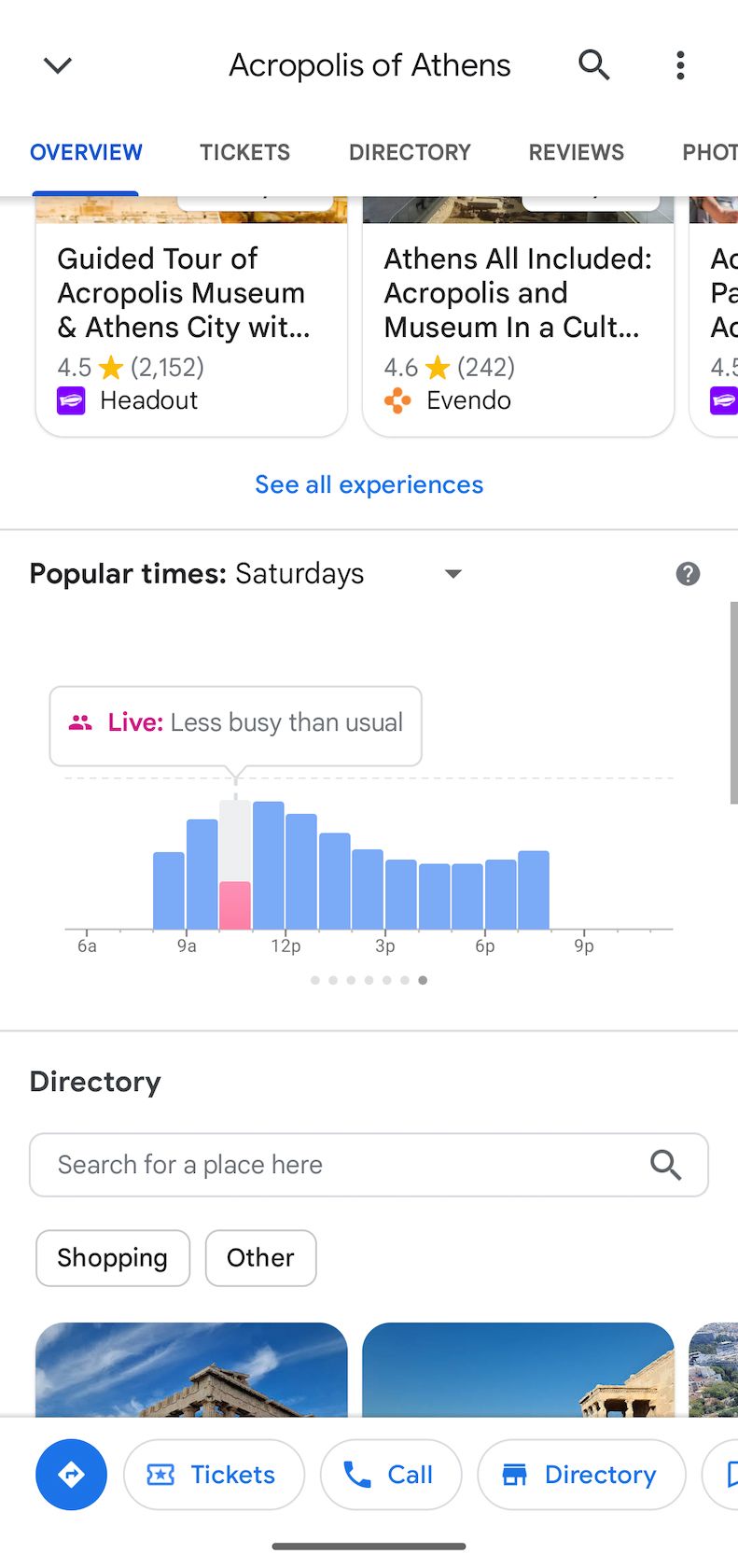In this mobile screenshot, you see a detailed view of search results for "Acropolis of Athens." At the top, a search bar with a magnifying glass icon on the right indicates the search query. Below the search bar, there are navigation tabs labeled "Overview," "Tickets," "Directory," "Reviews," and "Photos." The "Overview" tab is highlighted in blue, while the others are in black.

Directly under this navigation, partially visible images serve as thumbnails for different informational website tabs. The first tab displays the title "Guided Tour of Acropolis Museum in Athens City," rated 4.5 stars from 2,152 ratings, and is attributed to "Head Out." The second tab, titled "Athens All Included, Acropolis and Museum in Occult...," has a 4.6-star rating from 242 reviews and is associated with "Evendo." A third tab is present but partially obscured by scrolling.

Below these tabs, a blue "See All Experiences" link is followed by a thin horizontal line. The next section labeled "Popular Times" features a dropdown set to "Saturday." A bar chart illustrates the site's busyness throughout the day, from 6 a.m. to 9 p.m., with peak hours around 9 a.m. to 12 p.m. and a slight rise again at 7 p.m. An indicator above the chart reads "Live" in pink and "Less Busy Than Usual" in gray.

Further down, another horizontal line divides the content. The "Directory" section features a search box with placeholder text "Search for a Place Here," and a magnifying glass icon. Below the search box, two outlined buttons labeled "Shopping" and "Other" are displayed. A glimpse of three images representing an outdoor area is visible, requiring further scrolling to view fully.

At the very bottom, a navigation panel includes icons and buttons: a blue circle with an arrow pointing to the right, a "Tickets" button, a "Call" button, and a "Directory" button, all written in blue font.